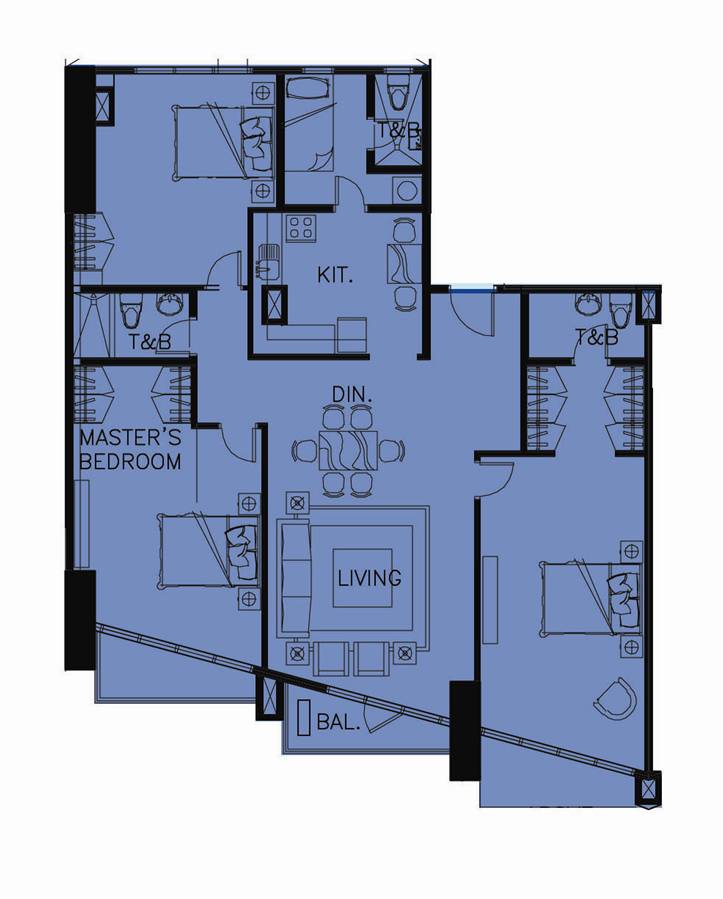A detailed floor plan of a home is depicted with black outlines against a white background. The rooms are shaded in a bluish color, providing clear differentiation. In the top right corner, the plan labels a room as "T&B," commonly referring to a Toilet and Bath. Below this, the room is marked as a kitchen. Adjacent to the kitchen on the right side, there is another "T&B," enhancing the property's convenience. Directly under the kitchen, a dining table is indicated, suggesting the dining area. To the left of the dining area, the map labels a space as the "Master's Bedroom," offering a prominent living quarter. On the far right of the plan, a living room is marked. At the bottom of the floor plan, there is a section labeled "BAL," referring to a balcony, providing outdoor access. Notably, there are thicker black rectangles, likely representing doorways or doors, adding to the structure's navigability.